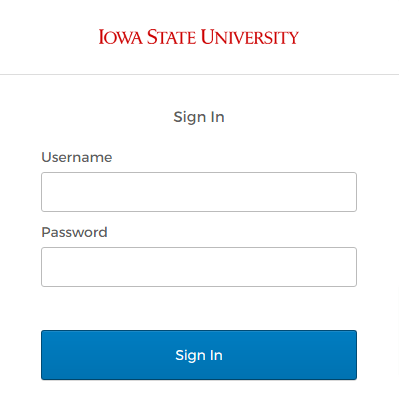The web page is designed with simplicity in mind, serving as a login portal for Iowa State University. At the top, in bold red capital letters and an elegant font, "IOWA STATE UNIVERSITY" stands out prominently. This heading is accentuated by a thin horizontal gray line directly beneath it. Below this line, the instruction "Sign In" is displayed in gray print, indicating the purpose of the page.

Centered on the page is a login form. The form consists of two white input boxes outlined in gray. The first box is labeled "Username" in gray text, followed by another labeled "Password." Positioned beneath these input fields is a large blue button containing the text "Sign In" in white letters.

The page offers no additional information about the specific application or service within the university that users are signing into. It is likely intended to be a central login gateway for students, faculty, and staff, granting access to their personal accounts once signed in.